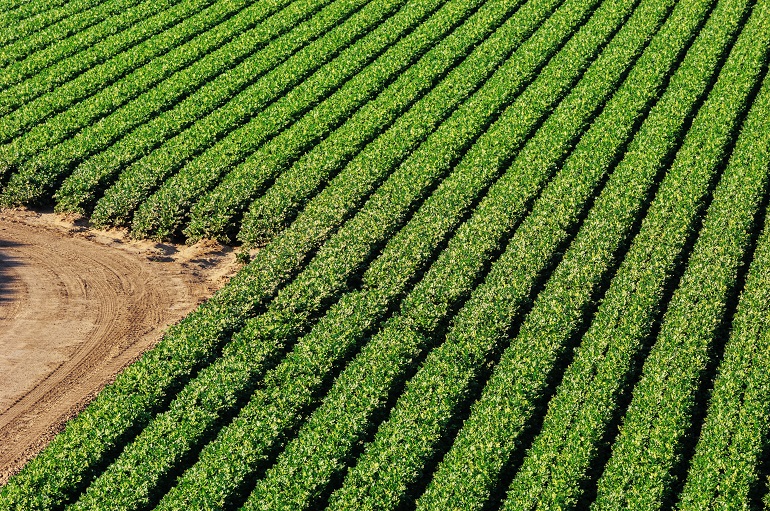This is an aerial photo of agricultural land featuring extensive rows of lush, vibrant green crops, possibly lettuce or a similar plant. The rows stretch from the bottom left of the frame towards the upper right-hand corner, creating a neat, repetitive pattern across approximately 80% of the image. Each row, about three to four feet wide, is separated by parallel black paths, forming a distinct line of demarcation between the crops. There are roughly 15 to 20 of these rows visible, running at a 45-degree angle right to left. On the left side of the image, there's a dirt road with visible tire marks, forming a 90-degree angle that cuts into the field, suggesting a path for vehicles or foot traffic along the edge of the farmland.